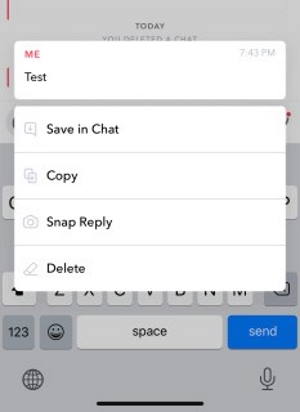The image depicts a phone screen with a gray main background overlaid by two prominent white rectangles, obscuring most of the content beneath them. The top rectangle prominently features the text "ME" in red letters on the left and "7:43 PM" on the right. Below this, the word "TEST" is displayed.

A slight break separates this from the second white rectangle, which contains four lines of text, each corresponding to different functions. The lines read as follows: 
1. SAVE IN CHAT 
2. COPY 
3. SNAP REPLY 
4. DELETE

The underlying main page is mostly hidden by these overlaying boxes but can be partially seen. At the top of this main page, the word "TODAY" is visible, followed by some blurred, partially covered text that is difficult to discern.

At the bottom of the screen, a keyboard is partially visible, covered mainly by the white rectangles. Despite this, you can identify some keys, including "123," a key with a smiley face, the space bar, and a blue "SEND" button on the far right.